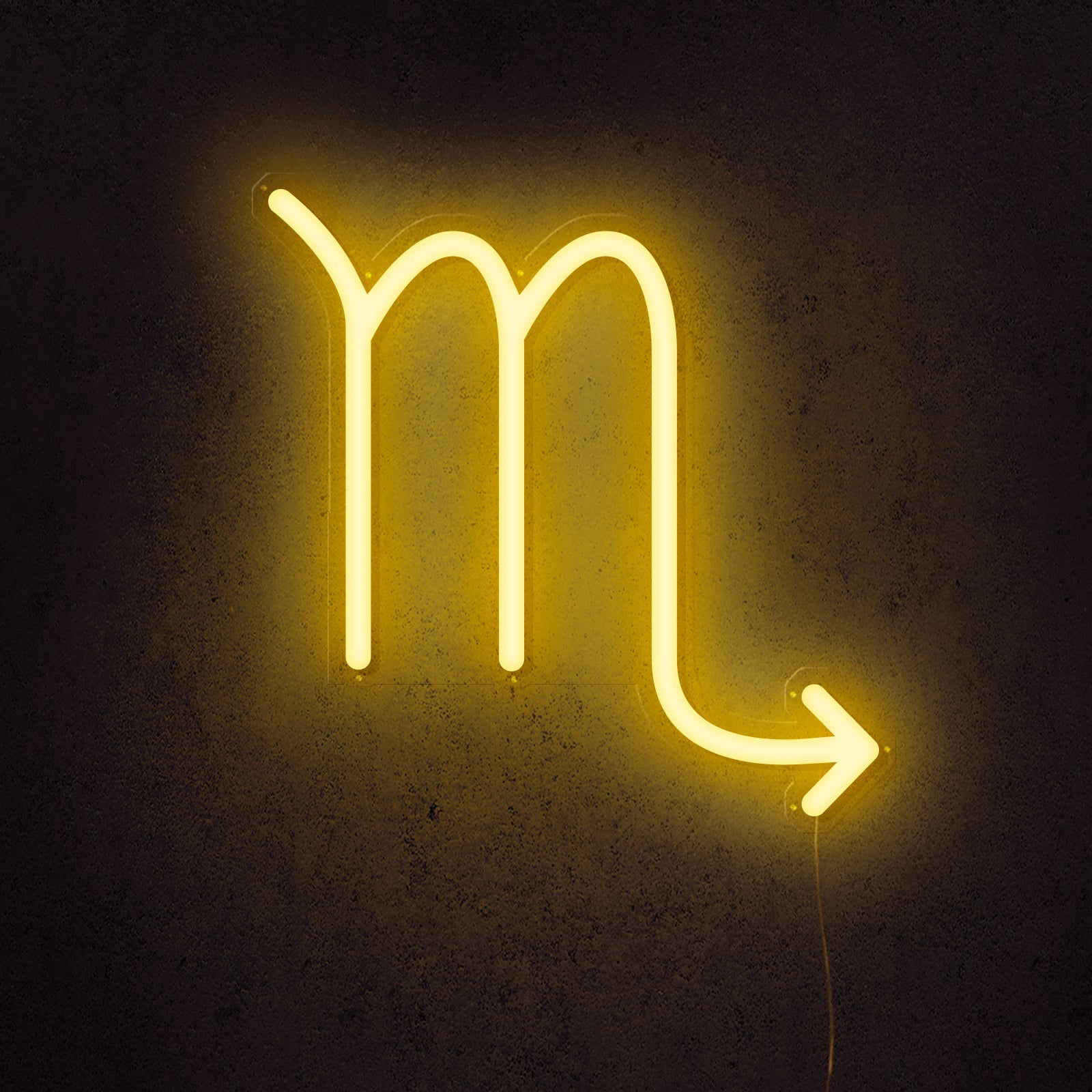This image features a neon "M" set against a pitch-black background, emitting a vibrant yellow glow. The "M" is designed with unique characteristics: the left side features a smooth curvature at the top, while the right leg extends downward past the alignment of the other portions. This right leg then transforms into an arrow that points to the right side of the image. Surrounding the neon letter is a hazy yellow aura, resembling wisps of smoke or mist emanating from the light. Adding to the visual intrigue, there is a drip effect originating from the arrow tip, creating a straight line that descends vertically to the bottom edge of the picture.